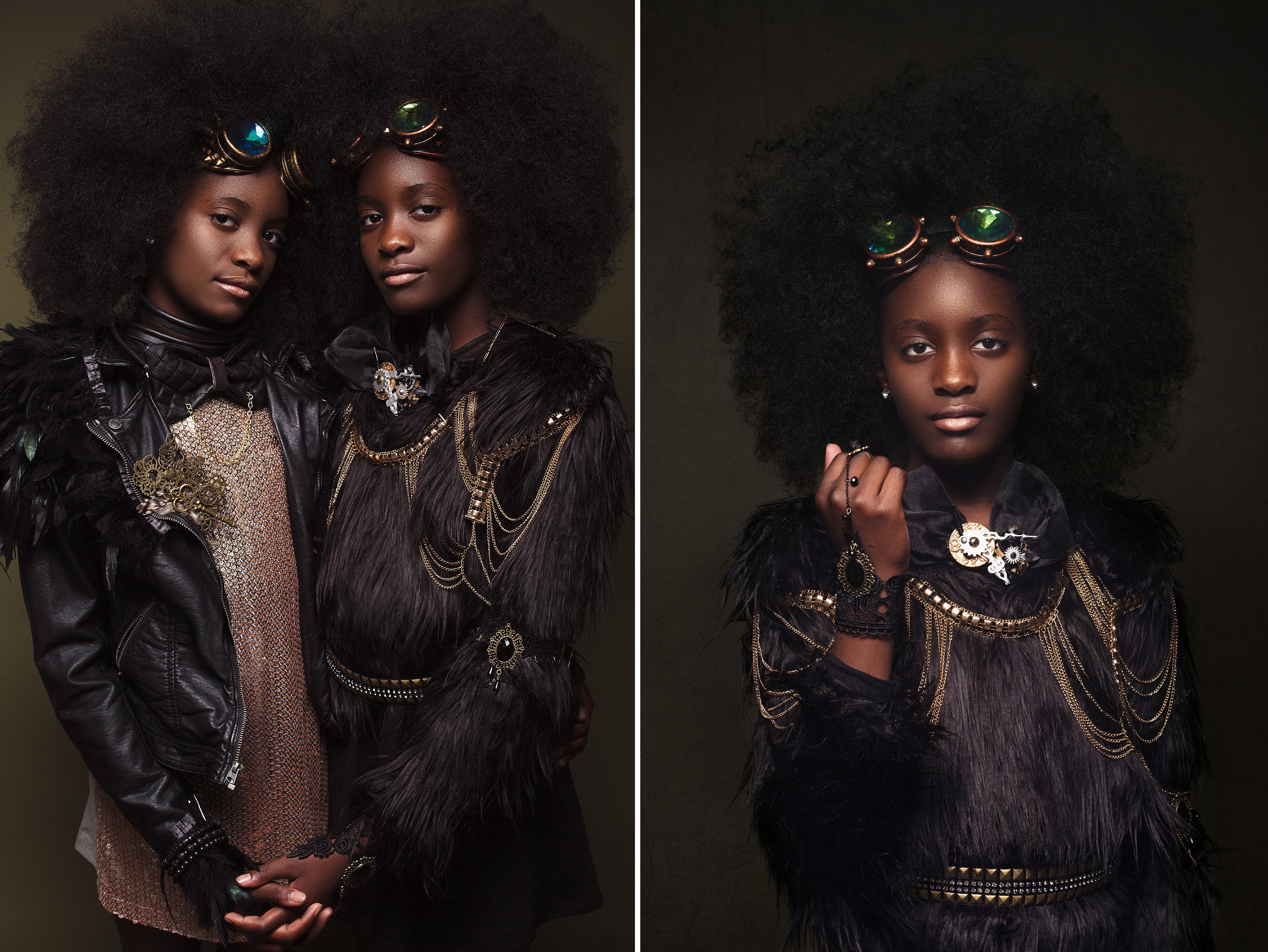This image is a side-by-side composition featuring two African American women adorned in elaborate steampunk attire. In the photo on the left, both women are holding hands and sporting voluminous afros, their hair extending about a foot in all directions, creating an impressive, fluffy halo effect. Each woman wears a distinctive pair of steampunk goggles on her forehead, the woman on the left with blue lenses and the one on the right with green. The woman with blue goggles is dressed in a leather jacket, while her companion in green goggles is dressed in a luxurious fur coat. Both women are accessorized with intricate steampunk jewelry that adds an extra layer of ornate detail to their outfits. 

The photo on the right focuses solely on the woman who was previously on the right. Here, she faces more directly towards the camera, showcasing her afro and green-lensed goggles more prominently. Her attire is the same fur coat from before, textured and stringy, giving the impression of a bearskin material. She wears an eye-catching large silver medallion necklace and a steampunk-inspired belt around her waist. The dark brown backdrop of the room accentuates the striking contrast with her large afro, emphasizing her elaborate and unique steampunk style.